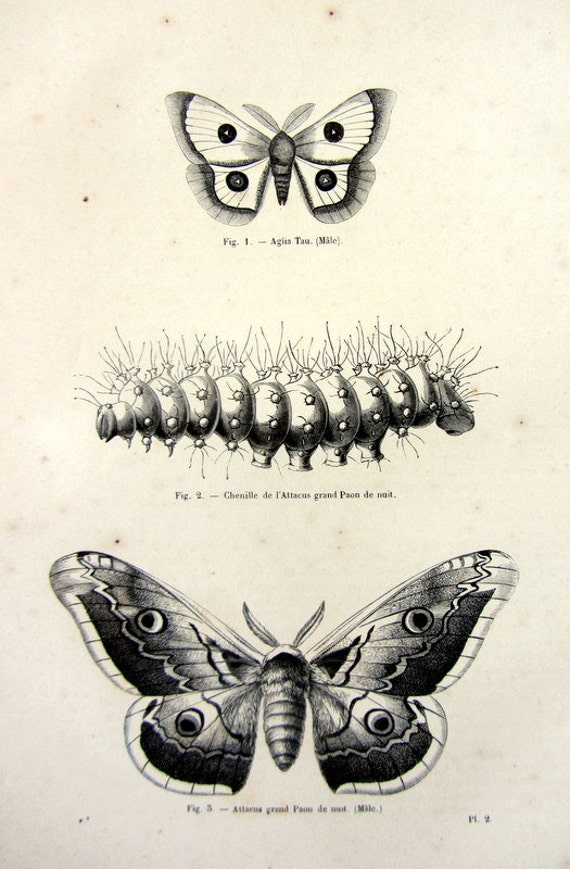This scientific illustration, rendered in a detailed and hand-drawn style using pen, pencil, or charcoal, depicts the various stages of a moth's life cycle. The drawing is set against cream-colored, parchment-like paper that suggests age or a classic style. 

At the top, marked as "Figure 1," is a small moth with feathery antennae. Its wings are primarily white with four prominent black spots — two on each wing — and black borders. Though labeled, the specific name is illegible. 

In the center, labeled as "Figure 2," is a caterpillar intricately detailed to show its segmented body and numerous spiky hairs. The caterpillar appears to have legs concentrated in the middle sections and is oriented to the right.

Finally, at the bottom, "Figure 3" showcases a fully-formed, much larger moth. This moth has a thorax in the middle, broad wings adorned with eyespots and horizontal stripes, and possesses a fuzzy body. The illustration is rich in detail and texture, emphasizing the contrast between the delicate upper moth and the more intricate and darker lower moth. A page number is faintly visible in the bottom right corner, reinforcing the illustration's scientific and archival essence.